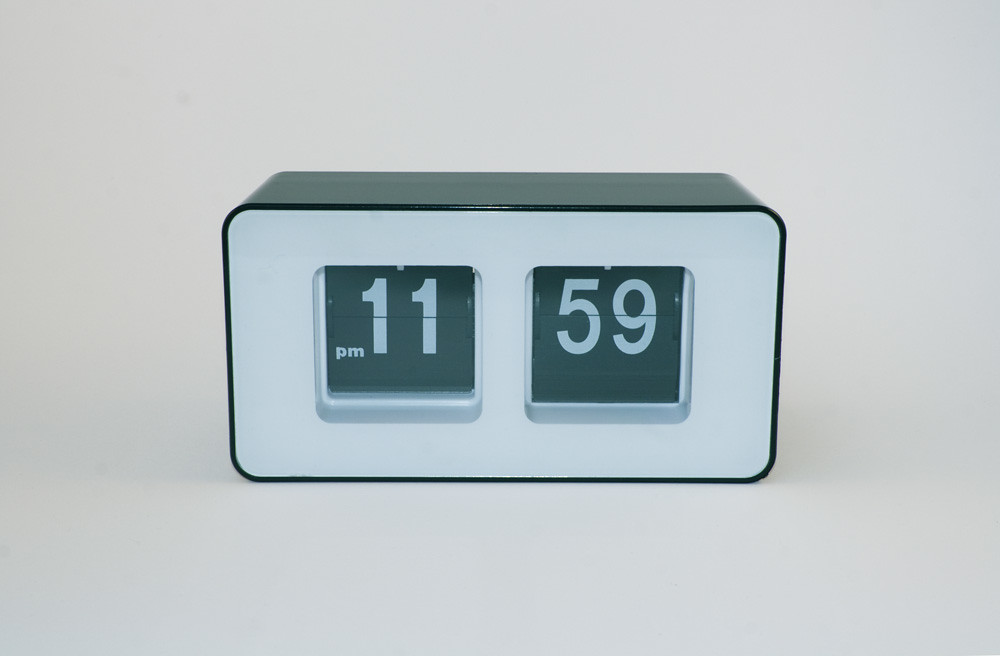This professionally shot image showcases a vintage flip clock against a pristine white backdrop. The clock, featuring a sleek rectangular design with smoothly rounded edges, has its front crafted from white plastic, while the sides are a contrasting black. The time displayed is precisely 11:59 PM, with the hours and minutes indicated by internal flaps that mechanically flip rather than using any digital displays. The flaps themselves are black, accentuating the bold, white numerals, and the "PM" indicator is prominently positioned to the left of the hour digit. The meticulous presentation highlights both the timeless design and the intricate functionality of this classic timepiece.